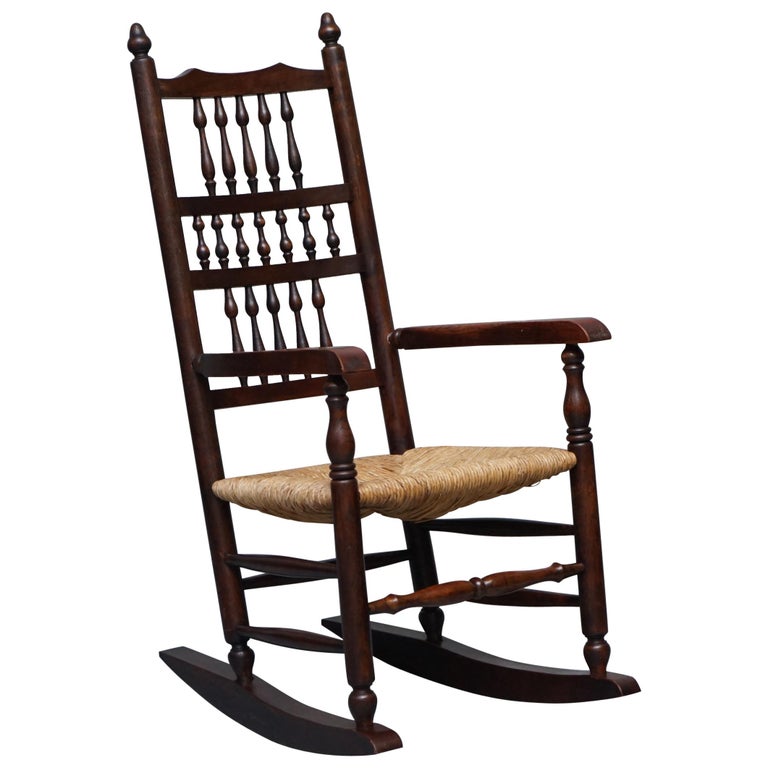This photograph showcases a classic wooden rocking chair, prominently featured as the sole object within the frame, emphasizing its details as a likely product image. The chair is crafted from dark brown wood and flaunts elegant spindle legs designed in a wider and shorter style which seamlessly blend into curved rockers at the base. The chair includes three rows of meticulously carved wooden spindles on its backrest. The top row features five taller, slimmer spindles, the middle row consists of seven shorter ones, and the bottom row mirrors the top with five slender spindles, all evenly spaced. At the apex of the chair, two rounded knobs add a decorative touch. The seat, created from tightly woven wicker or rattan, appears sturdy and well-maintained, with a light tan hue that contrasts with the dark wood. Horizontal crossbars connect the front and rear legs and additional bars connect the sides, bolstering the chair's structure. The design boasts bulbous details at its corners, adding to the overall vintage charm of the piece.